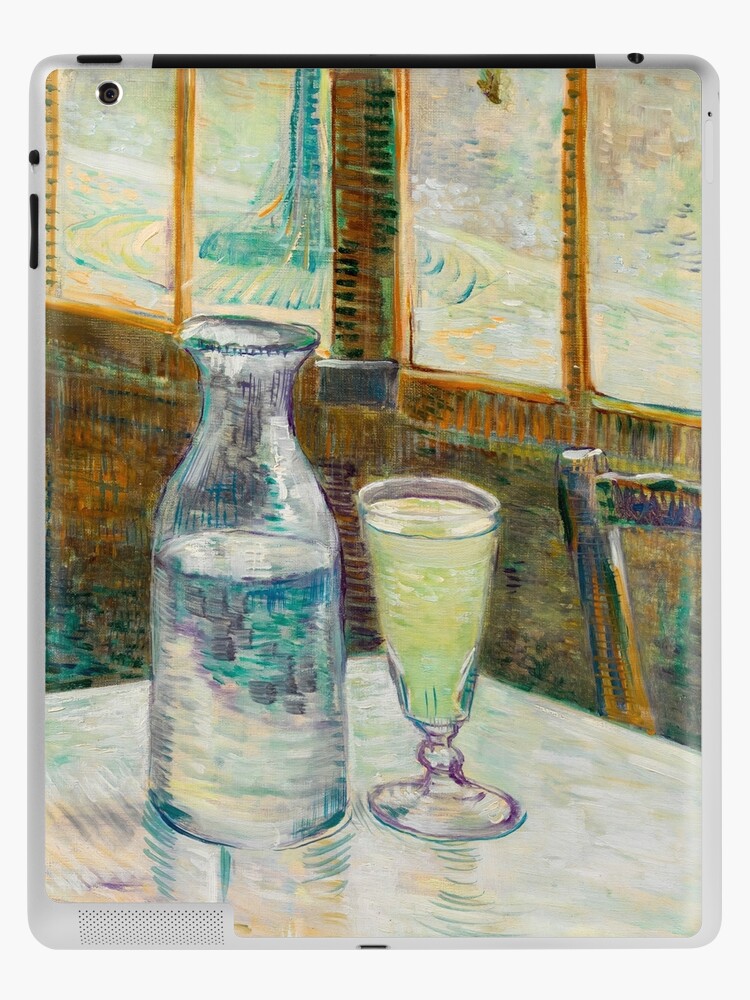The image depicts an oil painting displayed on the screen of a tablet, identifiable by the white, smooth perimeter with rounded corners, and visible tablet features like a speaker at the lower left, a camera lens at the upper left, and a USB-C input in the bottom center. The painting, reminiscent of Van Gogh’s style, likely portrays an interior scene, possibly a café or a room with a table in the foreground. On the table rests a cylindrical glass filled with a yellow liquid resembling lemonade and another footed goblet containing clear liquid. The table, painted with streaks that imply reflections, appears clear gray. To the right of the table, the top edge of a wooden chair is visible. The background reveals a light brown wall adorned with open windows, letting in ample light. The scenery through the windows is abstract, displaying an array of smudged colors like light orange, purple, green, and hints of blue, possibly indicating trees or outdoor objects in an impressionistic style.